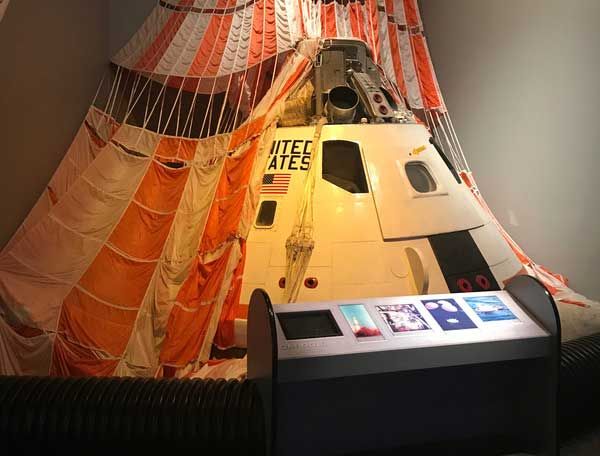The image depicts a detailed photograph of an old, conical space capsule that appears to be part of a museum exhibit. The capsule, which has “United States” and an American flag painted on its side, is likely from a NASA space expedition and is designed to splash down in water after a mission. It features a white exterior with a slightly tattered red and white striped parachute draped over it. Unique window placements and a sliding door can be seen, along with some intricate silver machinery protruding from the top.

The capsule sits behind a low protective wall, and in front of it, there's an illuminated display panel with black sides. This panel includes multiple rectangular sections—some containing photographs that appear to show images like birds, potentially a toucan, and scenes from space missions such as parachute deployments and splashdown recoveries in water. One of the rectangles on the display is notably empty. This detailed setup, along with the blank white wall in the background, accentuates the museum setting, suggesting a focus on educating visitors about space exploration history.